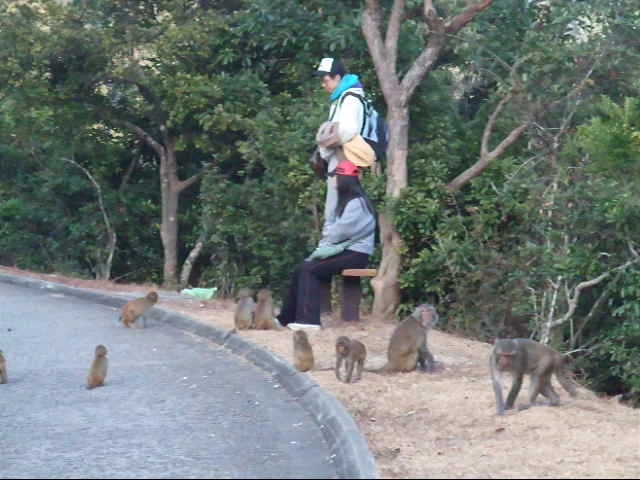In this detailed and vibrant image, a couple, a man and a woman, are positioned on a bench amidst a lush, green park or wildlife setting. The man, standing on the bench, wears a blue and white ball cap, a white sweatshirt with a blue hoodie underneath, a blue backpack, and presumably holds an item attached to it. The woman, seated on the bench, sports a red cap, a gray sweatshirt, black pants, and carries a green purse, complemented by her long, black hair.

Surrounding the couple are approximately nine monkeys, including two older ones and seven younger ones, some of which stand and gaze at the couple, while others meander about. The scene is set against a backdrop of dense, verdant trees with visible trunks, suggesting a rich, forested area. To the left of the bench extends an older paved road, accompanied by a dirt path adjacent to it, underscoring the natural yet slightly developed landscape. The numerous playful monkeys and the couple's attentive stance towards them add a lively, engaging dynamic to this tranquil setting.